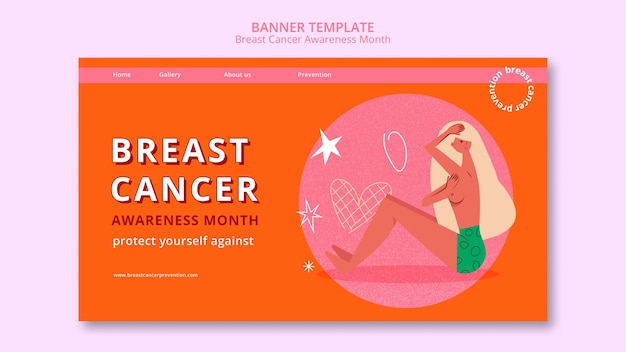This image is a screenshot of a banner template designed for Breast Cancer Awareness Month. The background features a greyish-pink tone, setting a subtle and respectful tone for the topic. At the top of the banner, the text prominently reads "Banner Template for Breast Cancer Awareness Month." Below it, an orange rectangle contains a pink banner header with white text displaying navigation options: "Home," "Gallery," "About Us," and "Prevention."

On the right-hand side of the banner, there's a pink circle with a white border that contains a cartoon illustration of a woman with long white hair. She is wearing green shorts or a very short skirt adorned with green circles and sitting on the ground. Her pose suggests a breast self-examination, as her left arm is raised, and her right hand checks her breast beneath her arm.

Within the pink circle, the background features various graphic elements: a shadow beneath the woman, a five-point star, a six-point star that isn't filled in, a heart with diagonal squares or diamonds, and a roughly drawn, incomplete circle. Her hair extends slightly outside the right edge of the circle, and elements of the shadow and stars spill over the left and right edges.

To the left of the pink circle, large white text with a brownish-red edge reads "Breast Cancer," followed by a smaller line of brown text stating "Awareness Month." Below this, in similar formatting, is the phrase "Protect Yourself Against," accompanied by what appears to be a tiny, illegible website address.

Additionally, surrounding the image are various smaller stars and shapes that enhance the visual appeal of the banner while emphasizing the theme of awareness and prevention.